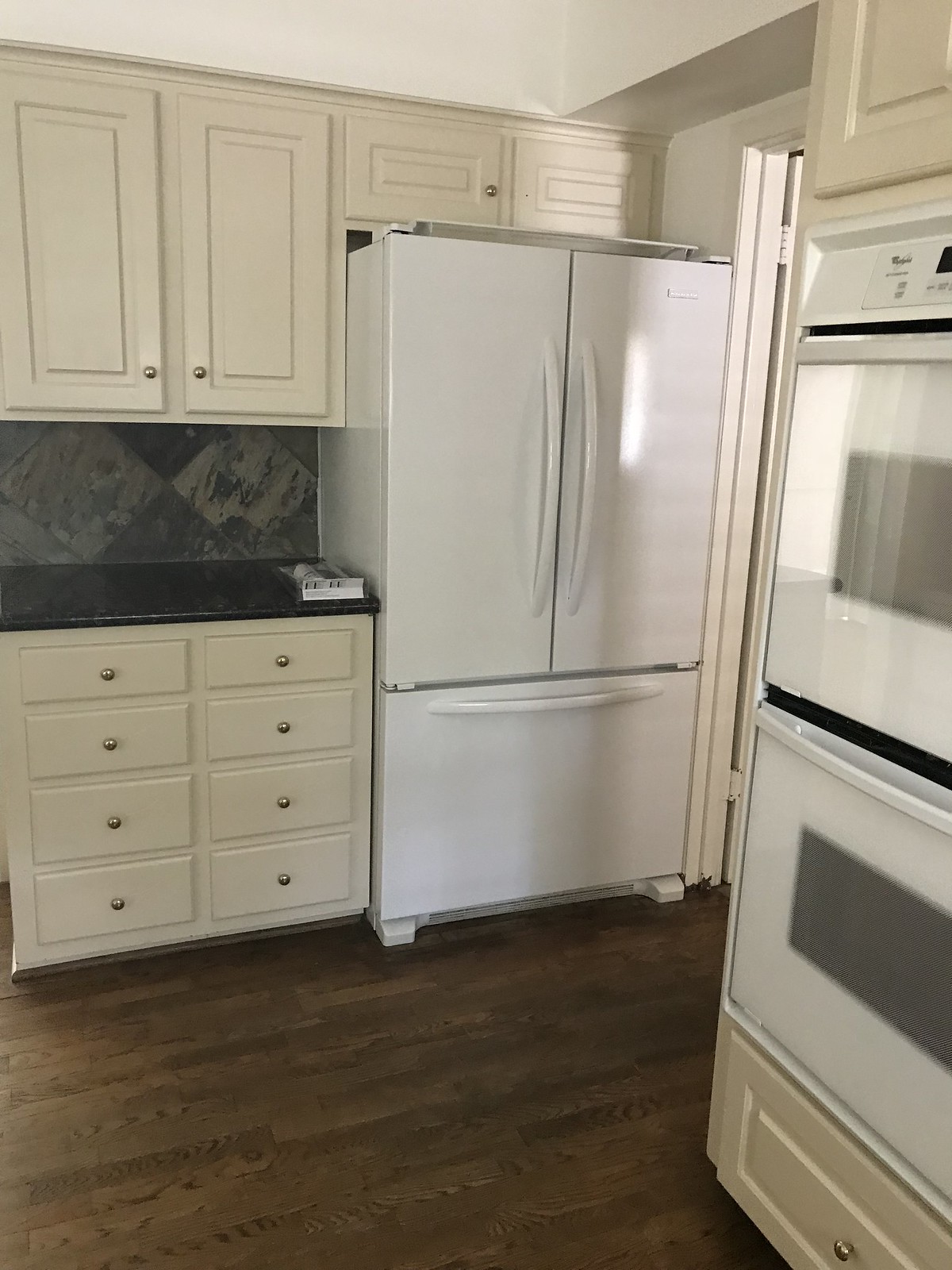The photo showcases a well-organized kitchen centered around a large white double-door refrigerator with a pull-out freezer drawer at the bottom. The refrigerator is positioned in the middle of the image, facing the camera, and features long vertical white handles on the upper doors and a horizontal white handle on the freezer drawer. Above the refrigerator, two small light brown cabinets are visible. To the left, there are two longer cabinets extending halfway down the refrigerator’s height, also light brown, equipped with gold handles. Below these cabinets is a blue wall section with a diamond or square pattern, transitioning into a dark marble countertop. The lower cabinetry matches the upper with light brown color and gold knobs, including two rows of smaller drawers.

The right side of the kitchen includes a white built-in oven with a clear glass window, and a second white built-in oven positioned below it, accompanied by another clear glass window. Beneath the second oven is a white drawer. Adjacent to the ovens, a small portion of a white dishwasher is visible alongside a doorway with light shining through, highlighted by its outline and trim. The flooring consists of dark brown wood, complementing the overall aesthetic of the kitchen.